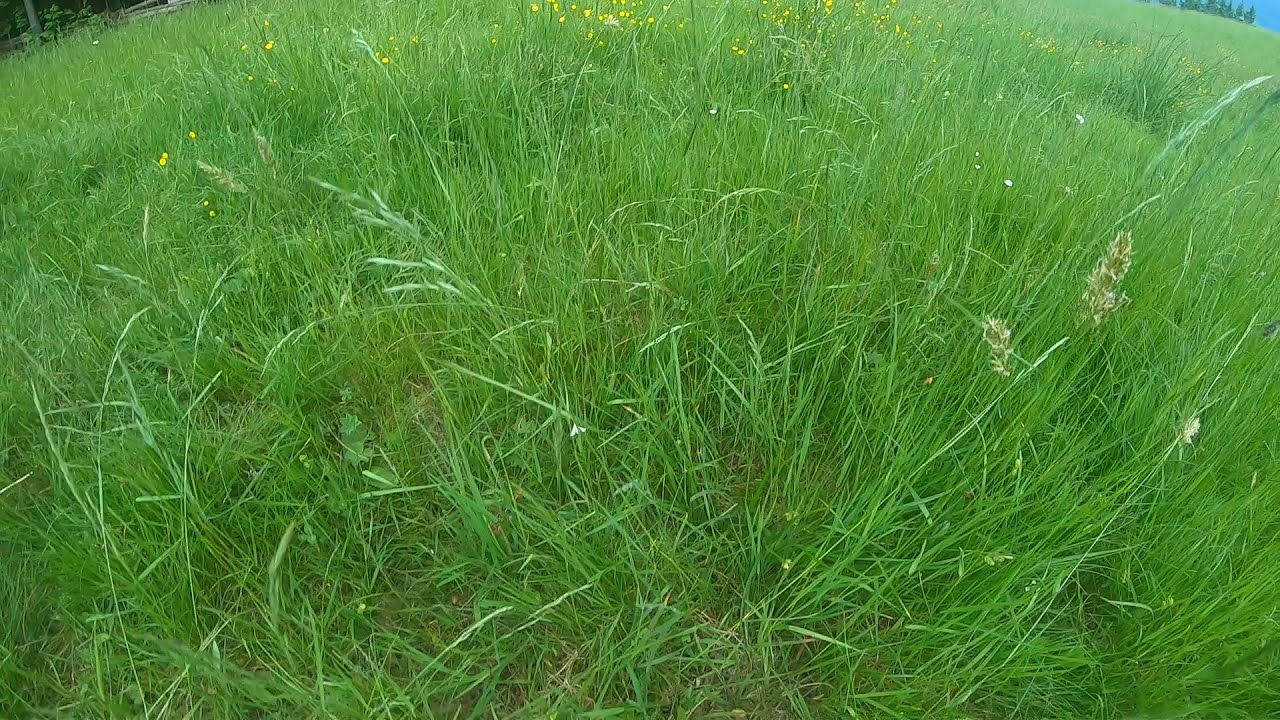This image captures a lush and wild field of long, green grass interspersed with various weeds and wildflowers. The photograph, taken with a fisheye lens, creates a curving, almost circular effect, pulling the viewer's focus towards the foreground while slightly distorting the edges. Predominantly green, the grass varies in lengths and types, with some areas showing spiky, budding weeds woven throughout. Yellow wildflowers are scattered sporadically, with notable clusters near the top edges and the right-hand side of the image. The field's wild, untamed nature is emphasized by its uniform greenery, though there is a small, slightly brown patch in the bottom center. In the upper right corner, a sliver of blue sky peeks through, while dark green woods are faintly visible in the upper left, providing a subtle backdrop to the predominantly earthbound scene. The overall atmosphere is one of natural, unkempt beauty, with soft, fluffy grasses and detailed weeds in the foreground, gradually losing detail towards the periphery.